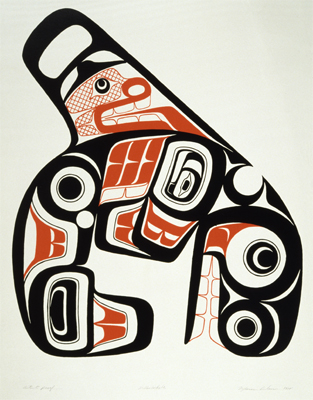The image depicts an abstract pattern featuring a prominent handle-like structure descending from the top left to the center, accompanied by an arch shape below. The entire pattern is outlined in black. At the top of the handle, there is a bird face adorned with a brown crosshatch pattern and a black cap. This bird face includes brown and black details, contributing to its intricate design. Below, the arch shape houses several black circular patterns and multiple instances of the letter 'B' printed in brown.

When viewed sideways, the pattern resembles a mask with mismatched eyes and a bottle-like neck capped at the top. The masked face below includes stylized features such as an orange mouth, which could be interpreted as an animal or a person, complete with three teeth on both the top and bottom. Behind the mouth, there is orange cross-hatching. Additionally, this section features an eye with a distinct white detail, adding to the ornate and highly stylized appearance of the piece. The artwork is a remarkable blend of abstract and representational elements.